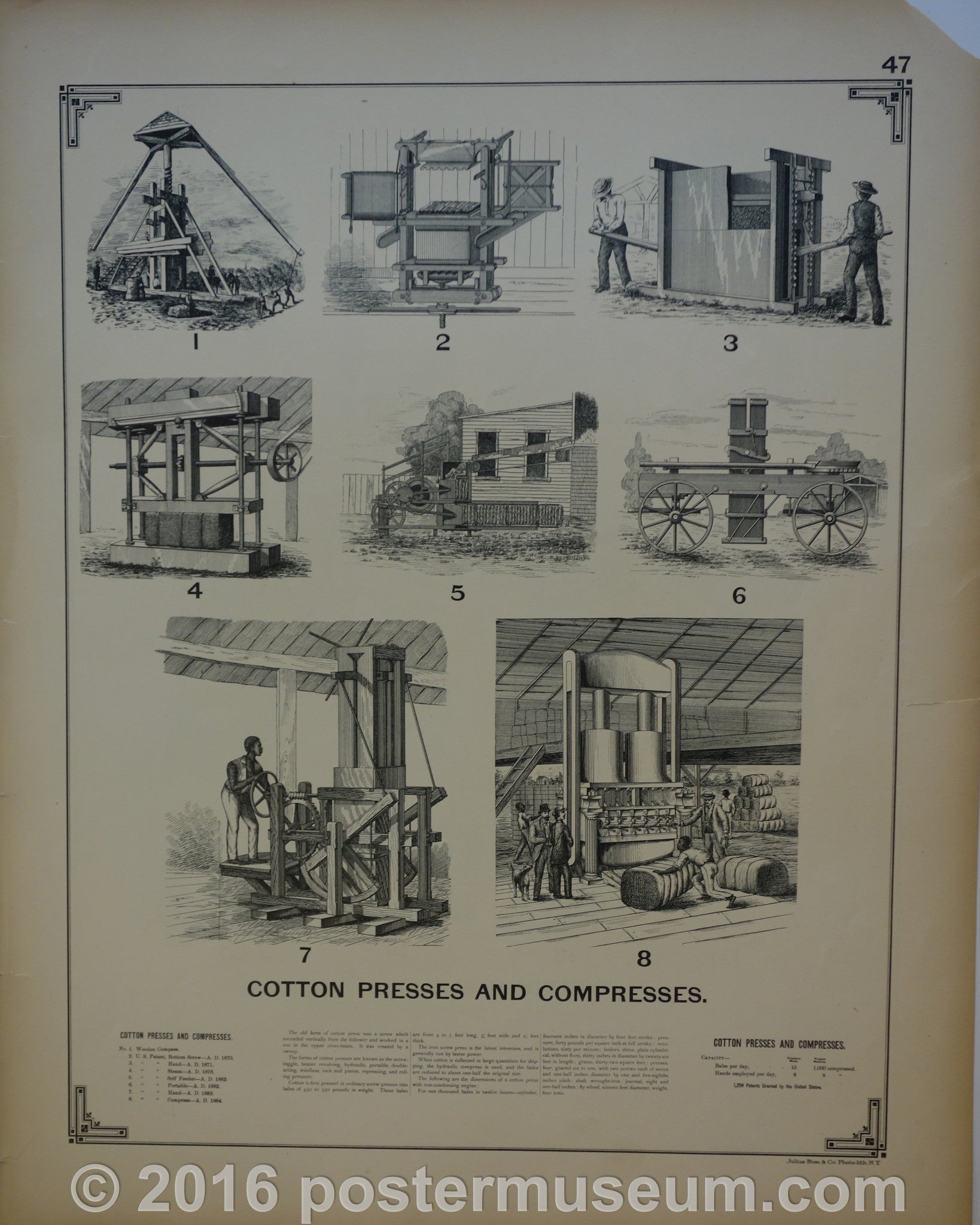This is a photograph of an old, black and white poster that appears to be from a catalog, specifically page number 47. The poster, printed on off-white cream-colored paper with aged edges, features eight highly detailed pencil drawings of mechanical equipment, each labeled numerically from one to eight. The drawings depict different cotton presses and compresses, showing increasingly elaborate machinery and people operating them. The bottom section of the poster prominently displays the text "Cotton Presses and Compresses" in large black font. Below the drawings, there's a small chart and three columns of fine print text offering further explanations, though the text is too small to read clearly. The entire poster is surrounded by a black border, and at the very bottom, there’s a watermark stating "Copyright 2016 postermuseum.com".